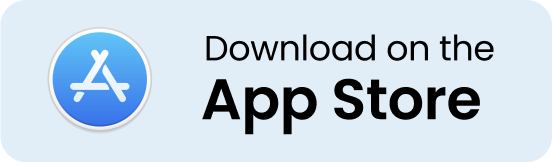This digital image features a minimalist design with a very pale blue background and a rectangular layout. Positioned to the left is a small circular logo, approximately the size of a nickel, outlined with a white border. Inside the circle is a stylized "A" created by intersecting white lines. Accompanying the logo, to its right, is text in two lines. The top line reads "Download on the" in a regular black font. Directly below, in bold black font, the words "App Store" are displayed, clearly separated into two words.